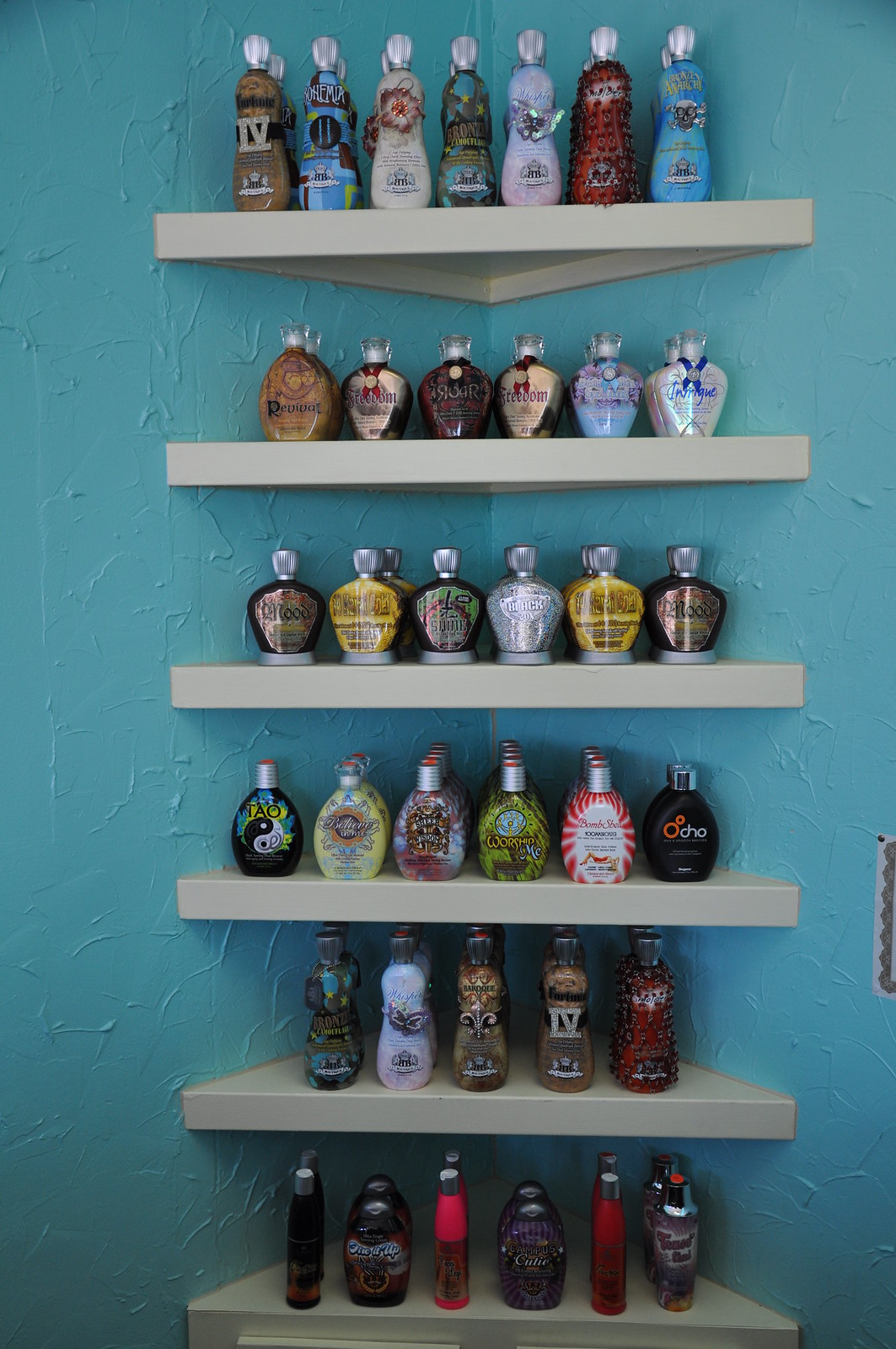The image depicts a corner of a room painted in turquoise blue, featuring six grey, triangular shelves that are evenly spaced and fitted perfectly into the corner. Each shelf holds an assortment of colorful bottles, likely cosmetics such as perfumes or shampoos, each differing in design. The topmost shelves display thinner, elegant bottles with ornate tops, resembling fancy alcohol or perfume bottles. The middle shelves contain more flask-like bottles, also in various colors, while the lower shelves feature smaller bottles, similar in size to protein drink bottles, also brightly colored. The bottom shelf holds a mixture of bottles, all in darker hues, maintaining the vivid aesthetic of the arrangement.